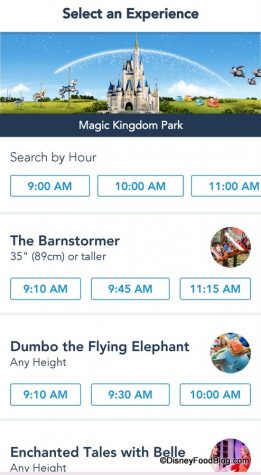This image is a screenshot from an unspecified Disney-themed app or website. At the top, the heading "Select an Experience" is prominently displayed. The central image features Cinderella's Castle, which could belong to either Disneyland or Disney World. To the left of the castle, two carousel horses are visible, while to the right, three flying elephant figures, resembling characters from Dumbo, soar in the air. A glowing, glittery, sparkly curved line arcs across the image, adding a touch of magic. Below, the text "Magic Kingdom Park" is shown along with a search feature labeled "Search by hour." Time slots listed are 9am, 10am, and 11am. Specific attractions and their details follow: "The Barnstormer" for guests 35 inches (89 centimeters) or taller with available times at 9:10am, 9:45am, and 11:15am; "Dumbo the Flying Elephant," accessible to guests of any height with slots at 9:10am, 9:30am, and 10am; and "Enchanted Tales with Belle," also for guests of any height. The bottom of the image is cut off, but a copyright notice by DisneyFoodBlog.com is visible in the bottom right corner. The image is oriented vertically, notably lacking any birds, automobiles, or motorcycles.